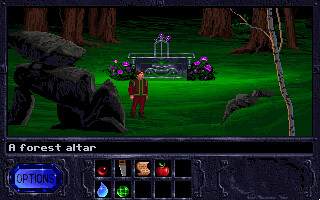This vibrant color screenshot from a retro-style video game captures a scene brimming with rich, bright hues and nostalgic pixel art. Dominating the top portion of the image, a lush landscape unfolds with bright green grass, giving way to a detailed forest backdrop. Central to the scene stands a distinguished altar, flanked by bursts of pink flowers. The altar itself is adorned with intriguing elements: three vertical objects crowned by two purple artifacts, suggesting a place of mystical importance. In front of the altar stands a valiant knight, clad in armor, seeming poised for action or in reverent observation. The background features gray boulders and towering trees, adding depth and texture to the scene. At the bottom of the screen, text identifies the setting as "A Forest Altar," grounding the viewer in the game's lore. To the left, a prominent blue button labeled "Options" invites interaction. Centrally positioned beneath the scene is a digital inventory, neatly organized like a cubby hole, displaying essential items such as an apple, a sword, and a drop of water, likely tools for the knight's quest. The overall image exudes a sense of adventure and fantasy, drawing the viewer into its captivating world.